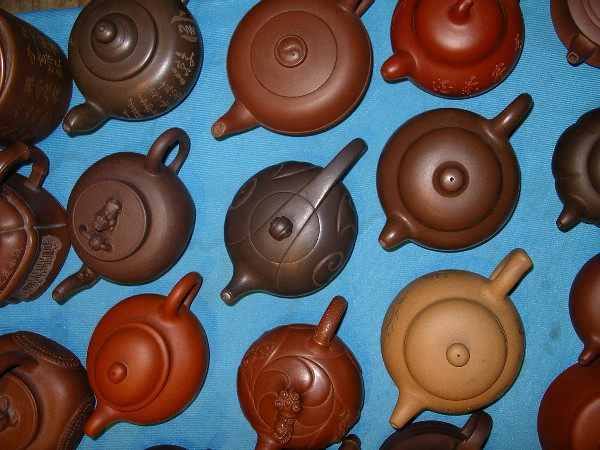This is a color photograph, likely generated or edited by AI, depicting an aerial view of small teapots arranged on a slightly textured, bright blue background that darkens towards the edges. The teapots, reminiscent of those found in Asian restaurants, vary in shades of brown from light khaki to deep reddish-brown. They are organized in vertical rows, with only portions of the outer rows visible due to the image's cropping.

The central row consists of a dark brown teapot at the top, a standard brown teapot in the middle, and an orange-brown teapot at the bottom. To the right, the row starts with a dark red teapot, followed by a dark brown one, and ends with a yellowish-golden teapot. The leftmost visible row shows two dark brown teapots and an orange-colored one at the bottom.

Each teapot has a circular lid design with several featuring smaller concentric circles in the middle. Notably, one teapot on the left has a decorative design instead of a plain circle, and another in the bottom center showcases an ornate, almost shell-like or floral top. Handles and spouts are visible on some teapots, suggesting a slightly varied perspective. There's a small wooden part in the bottom left corner of the image, and a potential blemish near the lower right corner.